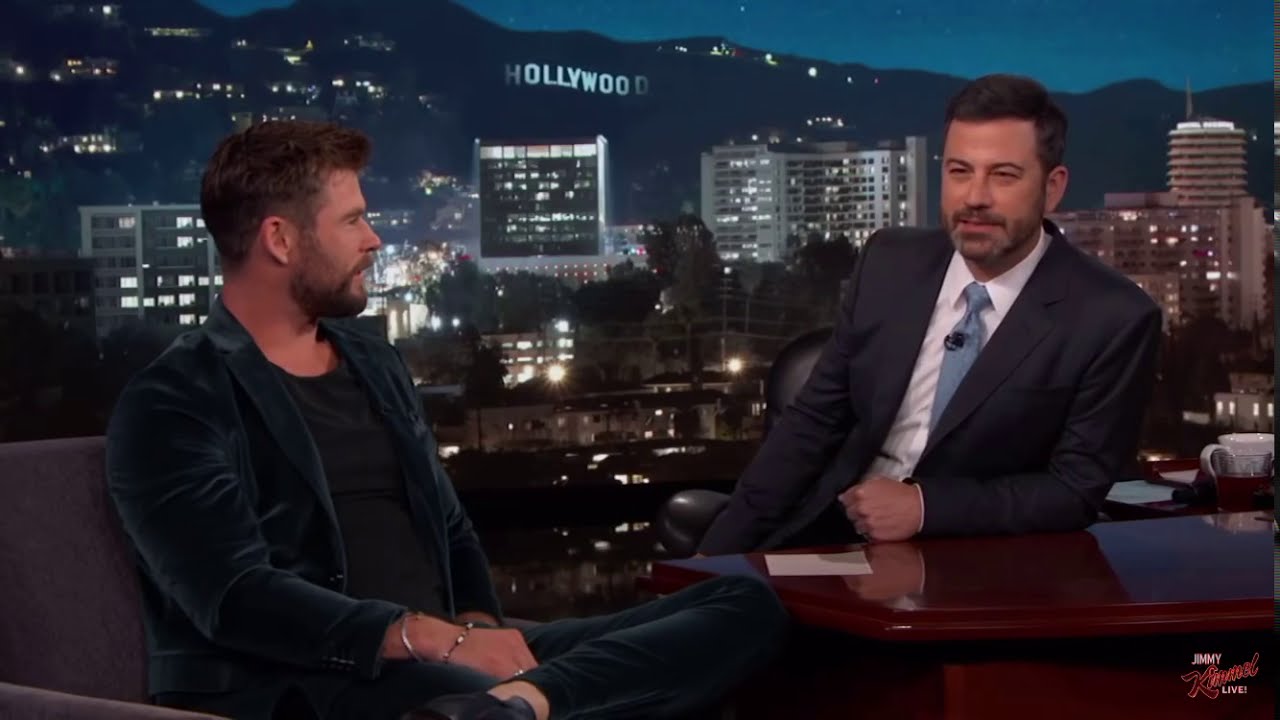In this detailed still image from the "Jimmy Kimmel Live!" TV show, the iconic Hollywood sign and a lit-up cityscape form the backdrop. Jimmy Kimmel, seated at a polished mahogany desk on the right, wears a sharp dark blue suit paired with a white shirt and a light blue tie. His elbow rests casually on the desk as he looks straight ahead, squinting slightly. To his left sits his guest, Chris Hemsworth, identified by his short brown hair, short beard, and mustache. Chris is dressed in a black and gray ensemble featuring a long-sleeved black jacket over a black shirt, with black pants and shoes. His leg is crossed, revealing an ankle adorned with bracelets. The "Jimmy Kimmel Live!" logo is visible at the bottom right of the image.